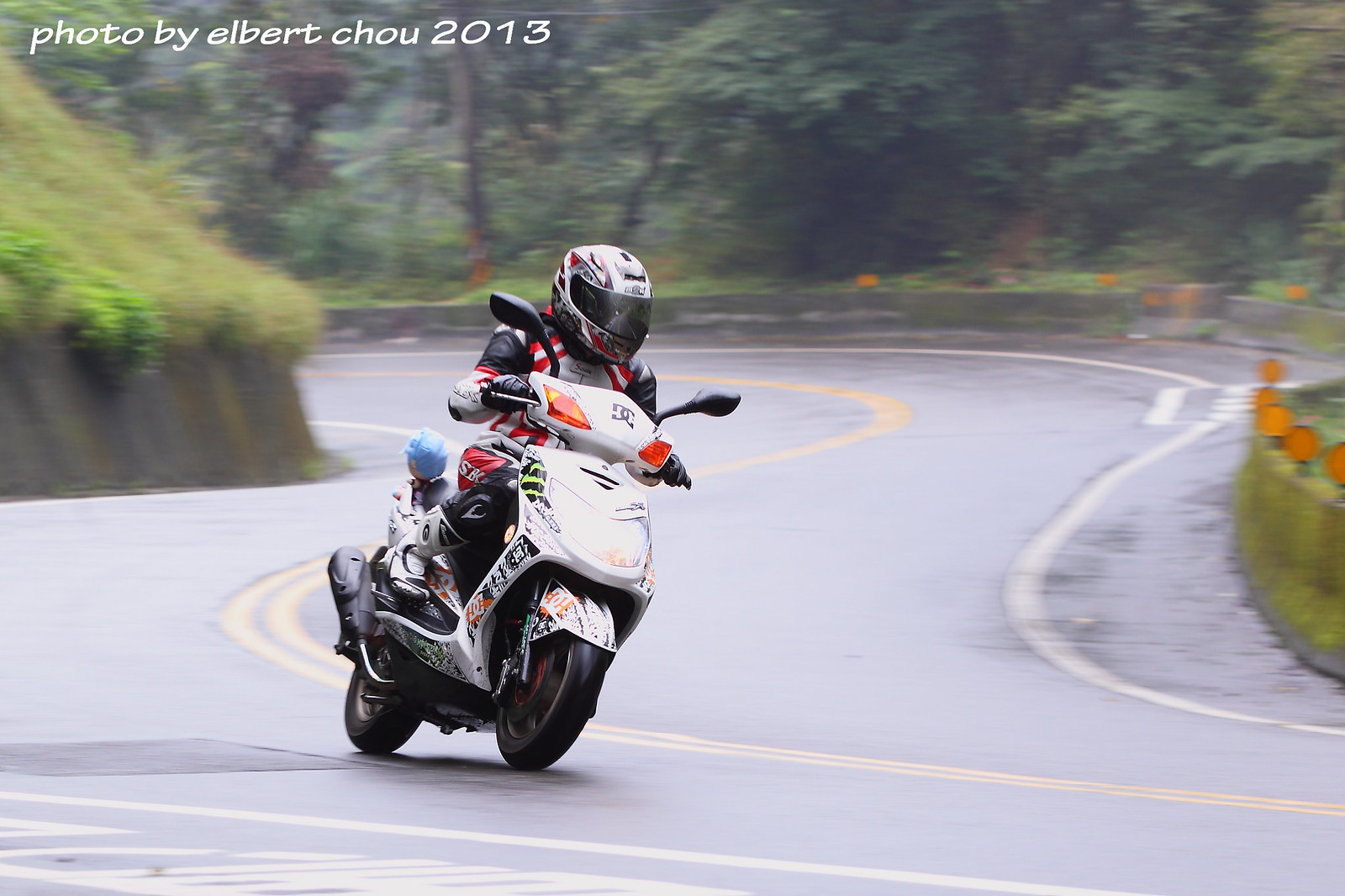In the photograph by Albert Chow, 2013, a person is captured riding a white and silver motorcycle adorned with various stickers, suggesting it might be a racing bike. The rider is outfitted in a striking red, white, and black suit and helmet, complete with a black visor, obscuring their face. The motorcycle is seen navigating a wet, curvy, two-lane road, marked by a double yellow center line and white edge stripes. The roadway is bordered by reflective lights and enveloped by a lush backdrop of large, green trees and verdant shrubbery. In the upper left-hand corner, the image is captioned with "photo by Albert Chow, 2013" in white lettering.